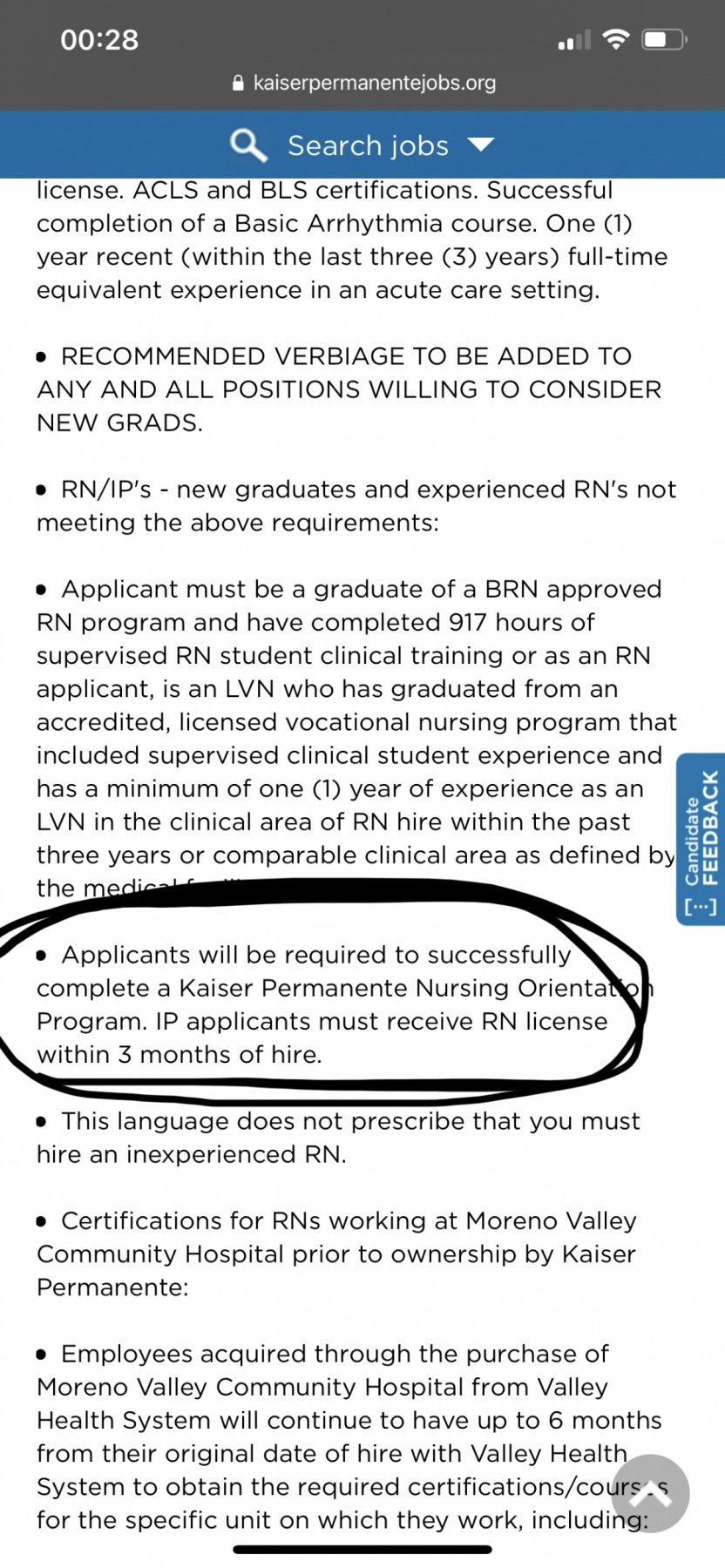This image is a screenshot taken from a mobile phone displaying a Kaiser Permanente jobs webpage. At the top of the screenshot, a gray horizontal banner spans across the screen, featuring the time "00:28" in white font on the left and the phone's signal strength, Wi-Fi status, and a half-charged battery indicator on the right. The central portion of the top banner contains a small white lock icon next to the text "Kaiser Permanente Jobs.org".

Below the gray banner is a blue horizontal banner with white font, featuring a magnifying glass icon beside the "Search Jobs" text, accompanied by a downward-pointing triangle, indicating a dropdown menu. 

The main section of the screenshot showcases a white background filled with blue bullet-pointed text detailing various job application requirements. Along the right side of the screen, the word "feedback" is prominently displayed vertically in blue font.

At the bottom of the screen, there is a transparent circle with an upward-pointing arrow, suggesting a user interface element for additional options or navigation.

One of the bullet points in the text has been digitally circled in an uneven, bold black outline, likely drawn by finger or pen tool. The circled text reads, "Applicants will be required to successfully complete a Kaiser Permanente Nursing Orientation Program. IP applicants must receive RN license within three months of hire."